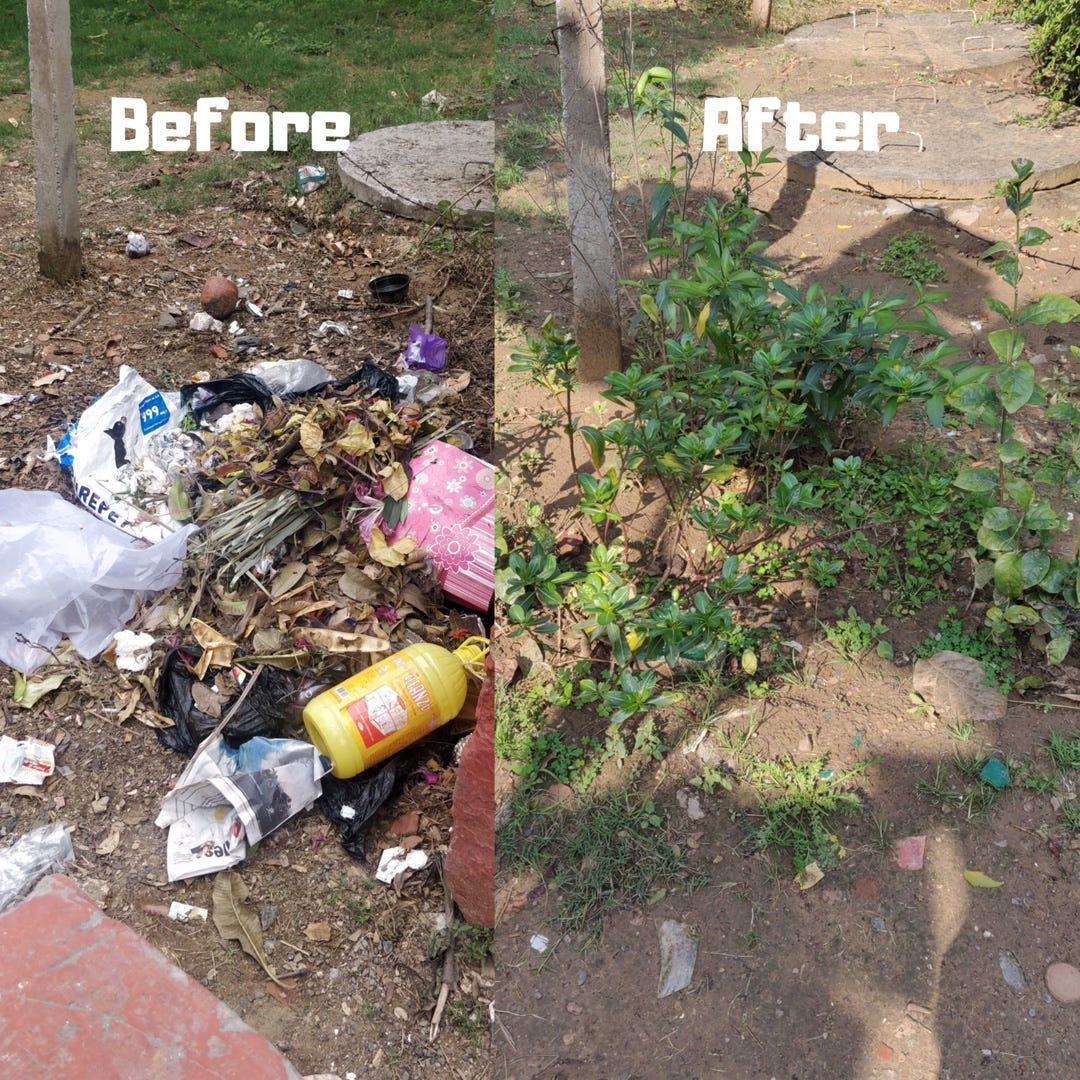This is a color photo compilation consisting of two side-by-side images labeled "before" and "after" in white text. The boundary between the images is not clearly defined. Both images capture a natural area resembling a park, with a stone cylinder or possible manhole cover in the background and a slender tree or wooden post in the upper left. The "before" image on the left is slightly narrower and is marred by debris, including trash, plastic bags, broken bottles, a yellow bottle, a white bag, and crumpled paper scattered among the brown leaves and dirt. The "after" image on the right shows a significant improvement: the trash has been cleared away, revealing dirt with a few rocks and sparse patches of green vegetation beginning to grow. Notably, a large red object appears in the lower left of both images, cut off in the "before" photo, and possibly made of stone. Overall, the comparison highlights an effort to clean up and rejuvenate the natural space, replacing litter with budding plant life.